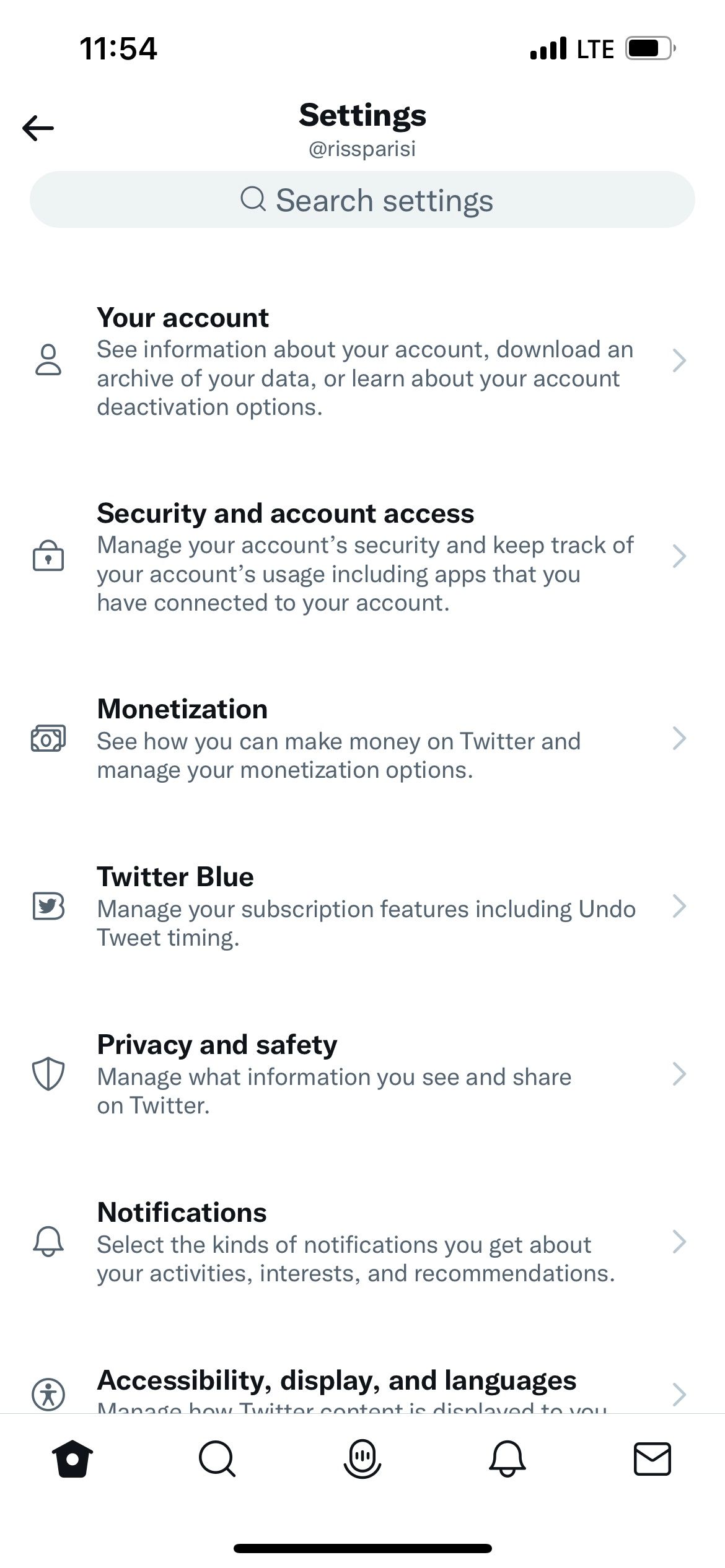A screenshot of a Twitter settings menu is displayed on a white background. At the top, the phone displays full LTE bars, a partially charged battery, and navigational icons such as a back arrow. Below, sections are listed with descriptive icons on the left and arrows indicating more options on the right.

1. **Security and Account Access**: A silhouette of a body with an arrow next to a padlock icon. This section allows you to manage your account security, track account usage, and oversee connected apps.

2. **Monetization**: Represented with a money icon. This section provides information on how to make money on Twitter and manage monetization options.

3. **Twitter Blue**: Indicated by a bird icon. Here, you can manage subscription features, including the timing for undoing tweets.

4. **Privacy and Safety**: Symbolized by a shield icon. It lets you control what information you share on Twitter and what you see.

5. **Notifications**: Marked by a bell icon. This section allows you to select types of notifications you receive about activities, interests, and recommendations.

6. **Accessibility, Display, and Languages**: Represented by a silhouette of a jumping jack figure within a circle. Here, you manage display settings, language preferences, and accessibility features.

At the bottom of the screen, a navigation bar displays a home button, search icon, microphone, bell, and an envelope. A black line runs across the middle of the screenshot, separating the upper and lower sections.